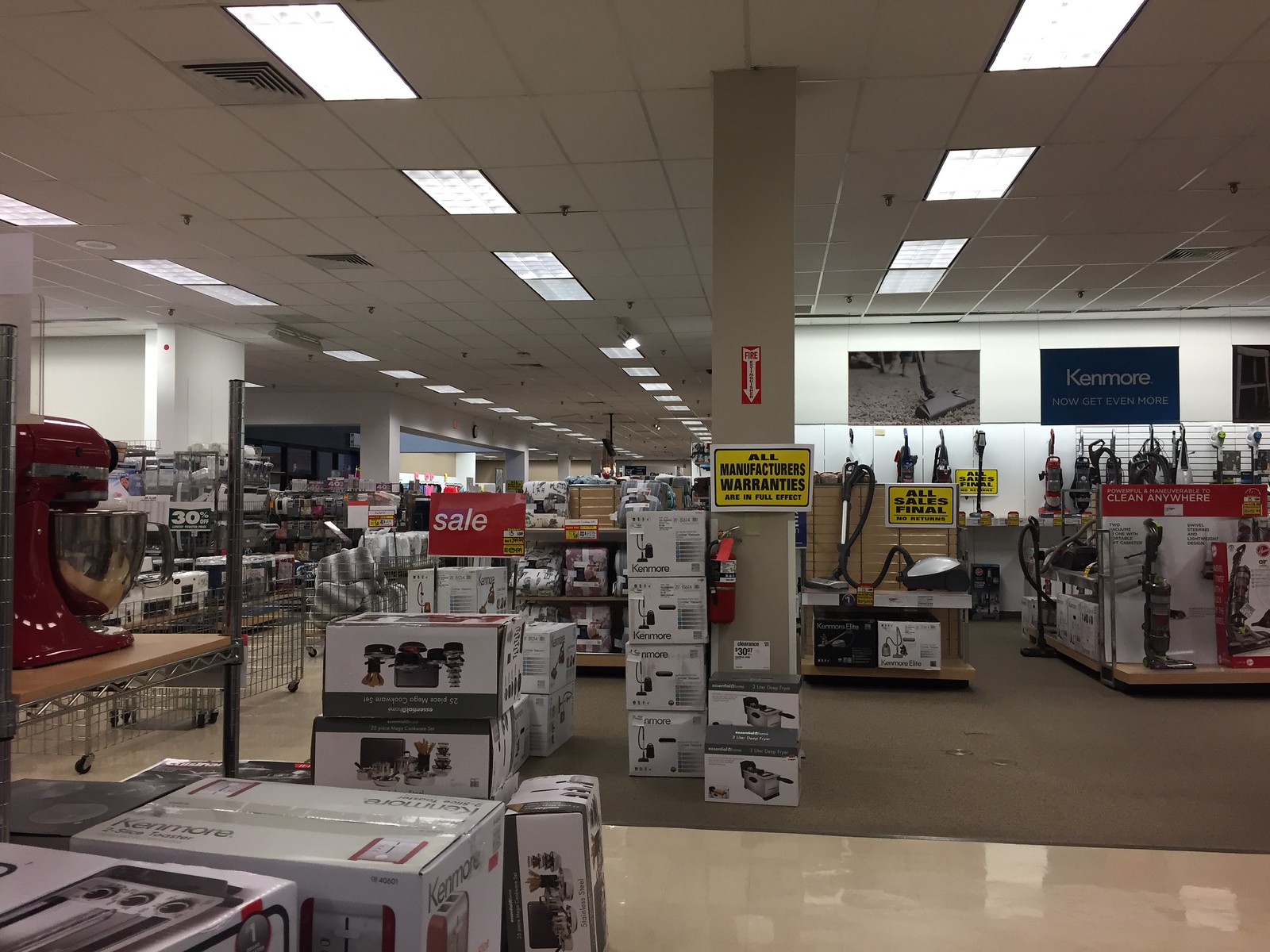In this detailed image of a large store, likely a department store such as JCPenney, Kohl's, or Target, the spacious interior reveals an organized array of home appliances. The ceiling features a grid of flush lighting, with rows of lights evenly spaced across the entire ceiling. The shiny floor reflects these overhead lights, adding to the store's bright ambiance. Several shelves and displays dominate the space, showcasing a variety of products.

Central to the display are numerous vacuum cleaners, prominently featuring brands like Kenmore, Dyson, and Dirt Devil. A distinct yellow sign with bold, black, all-capital letters reading "ALL SALES FINAL" is visible near a circular vacuum cleaner with its hose attachment. Another notable yellow sign indicates that all manufacturers' warranties are still in full effect. A Kenmore promotional sign, featuring white letters on a blue background, proclaims "Now get even more," accompanied by images of the vacuum in use.

Nearby, a red KitchenAid mixer, likely a 4.5-quart model, stands out amongst kitchen appliances, which also include a toaster oven and pots and pans. Some of the boxes, particularly those containing kitchen appliances, are stacked on shelves and even on the floor, with some visible upside down. A red sales sign announces a 30% discount on an assortment of items, including gray and white pillows or cushions in the distance.

Against one wall, vacuum cleaners are mounted on shelves, while other freestanding models, including a red vacuum, a gray vacuum, and a handheld vacuum, are positioned in front. Adjacent to a white pillar, which bears the "All Manufacturer Warranties" sign, a fire extinguisher is prominently displayed, enhancing the practicality and safety measures within the store.